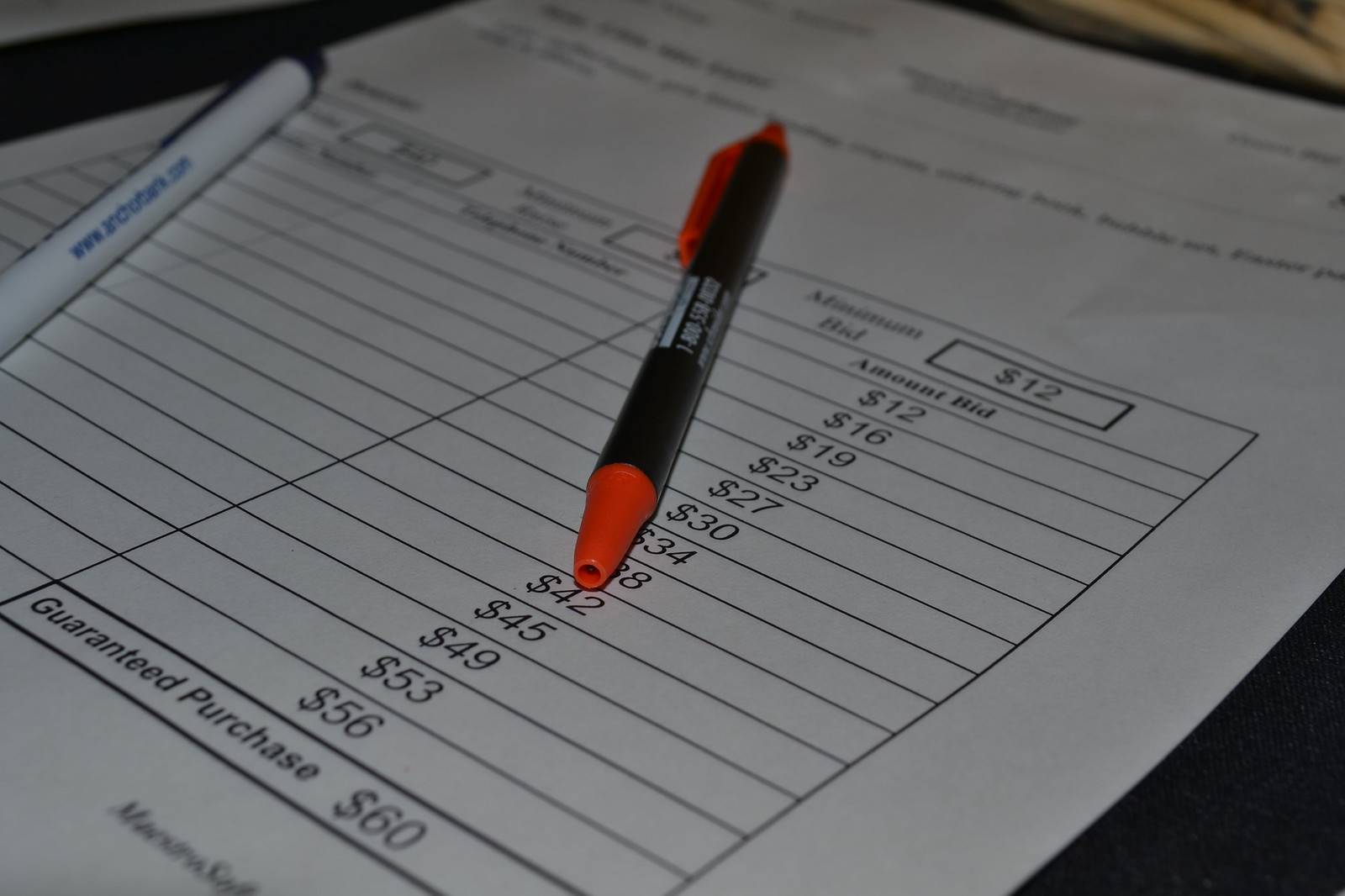The image shows an indoor photograph of a ledger page laid diagonally from the lower left to the upper right on a black background. The top third of the page contains blurred text that is unreadable, while the bottom two-thirds feature a detailed table. The table has three columns, although the contents of the first two columns are unclear due to the image angle. The third column, labeled "amount bid," lists a sequence of bid values: $12, $16, $19, $23, $27, $30, $34, $38, $42, $45, $49, $53, and $56. At the very bottom, within a bolded black-framed box, are the words "guaranteed purchase $60." At the top of the table, there are three smaller boxes, with the rightmost box indicating "minimum bid" of $12.

Two pens are placed on the ledger. One pen, centrally positioned, has a black body with orange tips and features a 1-800 number in white print. The other pen, partially visible at the top left corner of the page, is white with navy blue detailing and displays a website address in blue font. The overall dimension of the paper appears to be approximately six inches wide and four inches tall, and there is a lighted area in the upper right-hand corner that is also blurred out.